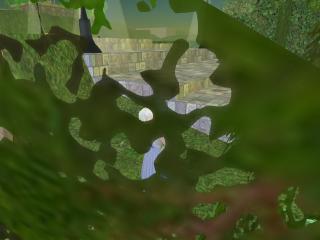The image is abstract and difficult to define, featuring a layered composition with several shades of green, gray, and touches of black and brown. The background appears mottled, creating a texture that resembles leaves or paper scattered on a water surface. One distinctive element is a white dot situated at the center. The image evokes the appearance of a dark green puzzle with cutout sections revealing lighter green and gray areas underneath, contributing to its enigmatic and abstract nature.